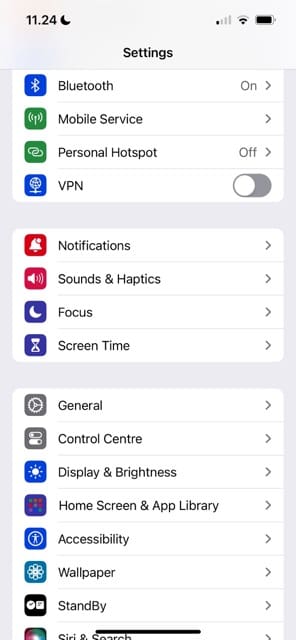The screenshot depicts the settings interface of a mobile device. At the top, the time is displayed as 11:24 PM, indicated by a moon icon, suggesting nighttime. The battery indicator shows a strong charge, while the signal strength appears weak. Centralized in bold is the heading "Settings."

Below the heading, standard icons are displayed to the left of their respective functions: Bluetooth is enabled, mobile service is active, Personal Hotspot is off, and VPN status is unspecified.

The settings are organized into sections. The first section includes: Notifications, Sounds & Haptics, Focus, and Screen Time. The subsequent section partially visible includes: General, Control Center, Display & Brightness, Home Screen & App Library, Accessibility, Wallpaper, and Standby. Additionally, a small portion of the "Siri & Search" option is visible at the bottom.